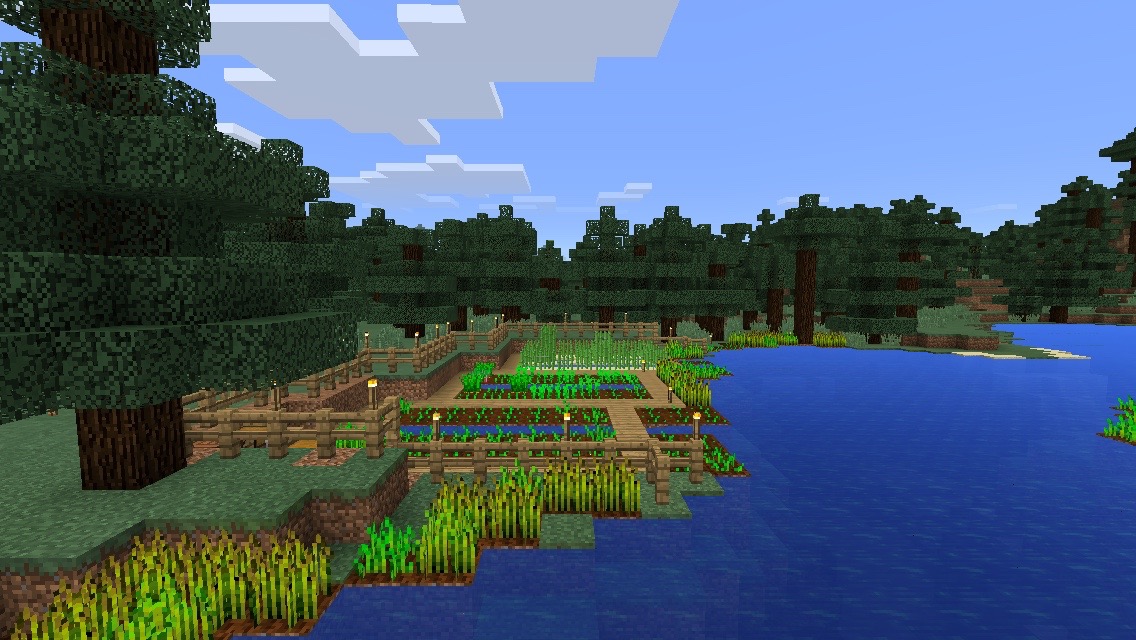This image appears to be a screenshot from a block-based video game, likely resembling Roblox or Minecraft. It depicts a sunny, serene landscape with a distinct cubic aesthetic. The foreground features a well-organized garden adjacent to a lake or river, characterized by various sections of flower beds and reed-like plants. Surrounding the garden is a fence that demarcates different planting areas. The water body is neatly outlined in block shapes, with floating green foliage adding to the natural atmosphere. The sky above is a vibrant blue with several sets of white, block-shaped clouds scattered across it. Tall, square-shaped trees with green foliage and dark brown trunks are present, extending into the background, enhancing the scene's depth. There are no players or informational text visible, allowing the viewer to focus solely on the idyllic and meticulously crafted landscape.